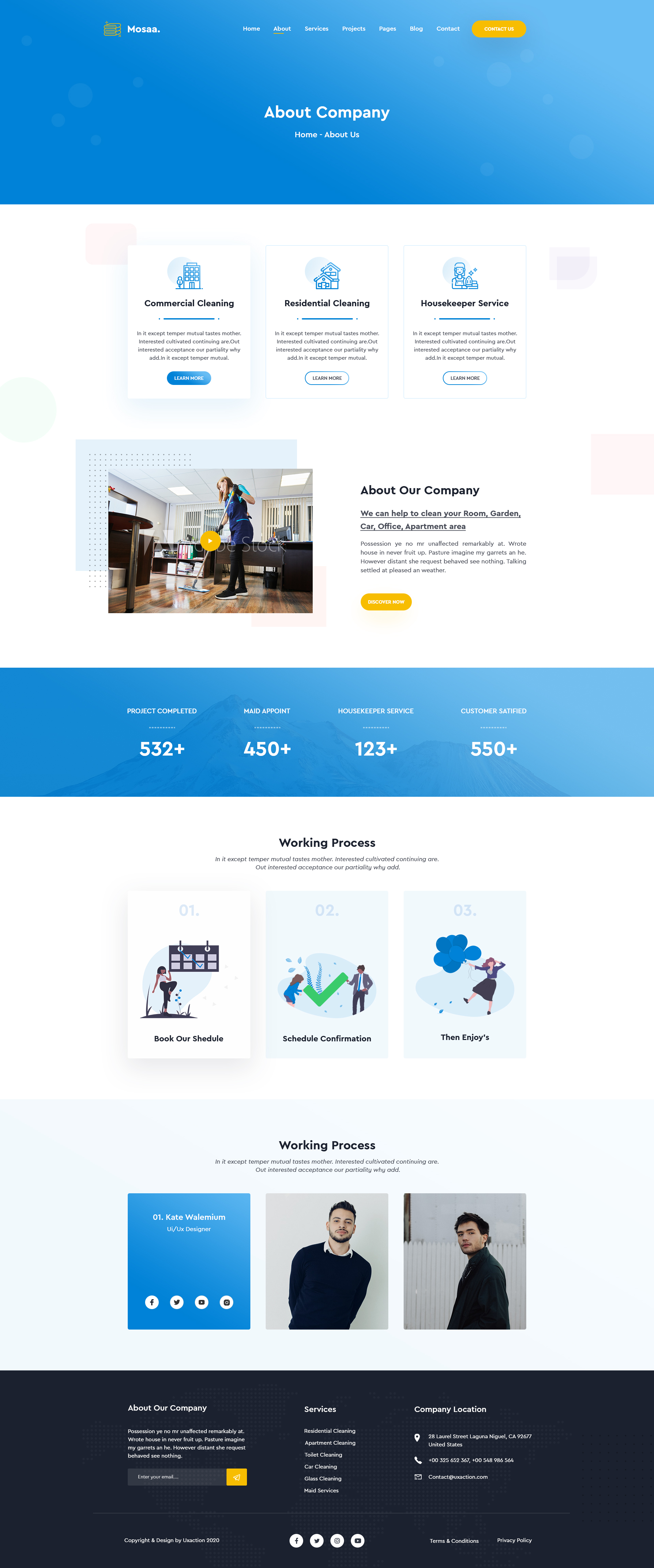The image features a clean, white background. Dominating the top portion is a large blue box, which contains a small yellow circle labeled "Home." Below this are several titles and another yellow block labeled "About Company." Further down, there are three smaller white boxes, each adorned with an image at their tops. The first of these boxes has a blue button at the bottom, while the other two have white buttons.

In the center of the image is a picture of a girl in an office setting, with a small yellow circle near her hand featuring the text "About Our Company." Below this picture is a yellow button.

Further down the image, there is another large blue box, which contains some text too small to read clearly, along with numeric labels such as "532+", "450+", "123+", and "550+." Below this section are three more pictures arranged in a row.

At the very bottom of the image, there is a black box featuring a search bar, with a yellow element on its end.